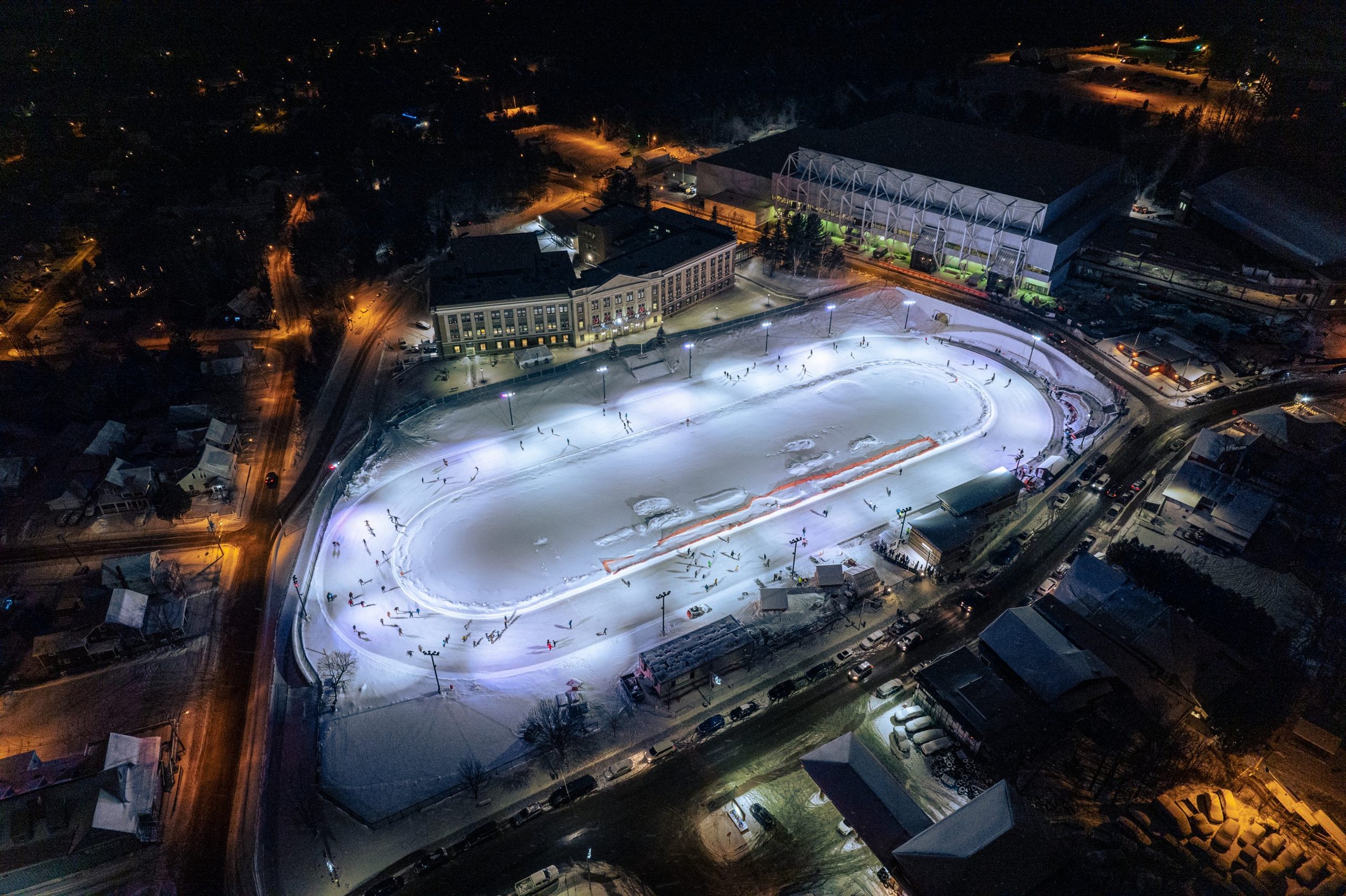This is an aerial photo taken at night, showcasing a stately classical building behind a large, stadium-style ice skating rink. The skating rink, brightly illuminated by floodlights around its edges, reveals skaters circling its perimeter, leaving the ice-covered center noticeably empty. The vivid surroundings feature city streets glowing with golden-orange sodium streetlights, interspersed with houses and additional buildings, adding a warm and inviting atmosphere to the nighttime scene. The shot, likely captured from 50 to 100 feet above, provides a sweeping view of the bustling, yet serene urban environment mixed with the lively activity of the skaters.